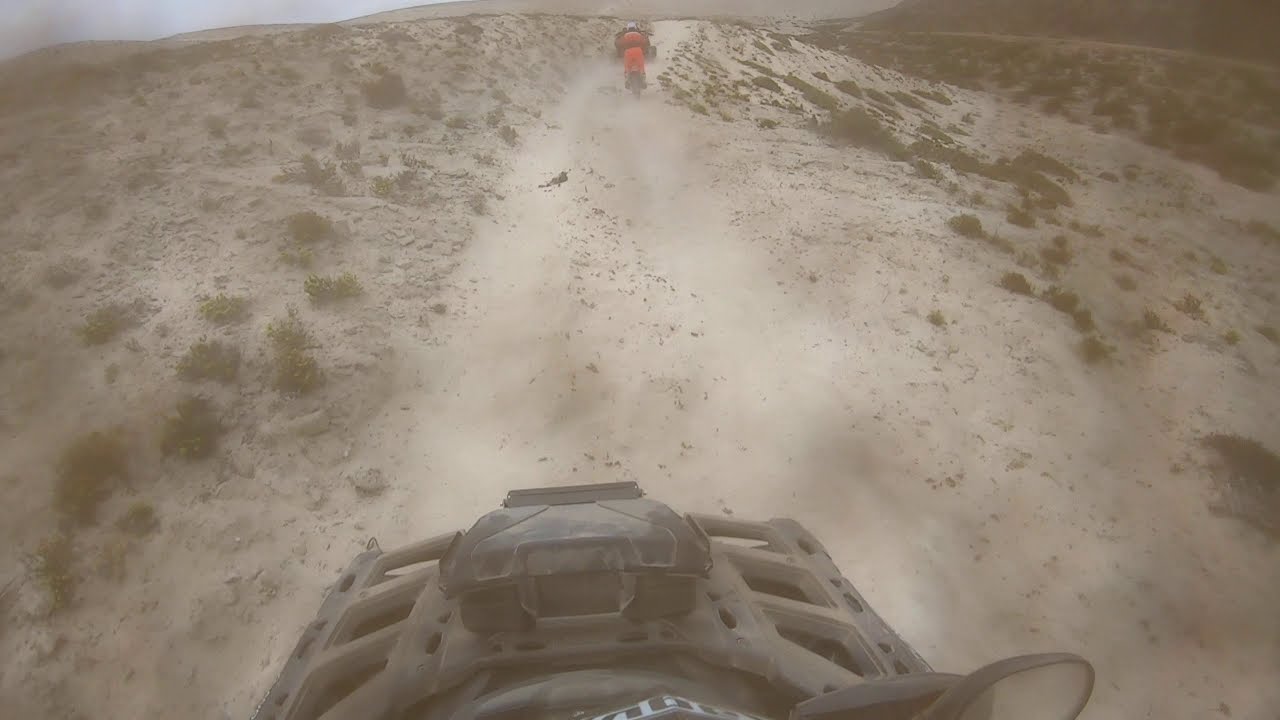The image captures a dynamic scene of an adventurous ride through a dusty, largely barren landscape. The foreground prominently features the front wheel of what appears to be a motorcycle or possibly a go-kart, caked in dirt and grime, emphasizing the rugged conditions. The ground itself is a mixture of dry dust and mud, dotted with sparse, dying greenery. In the distance, a man clad in a red outfit rides another vehicle, either a dirt bike or a similar machine, adding a sense of companionship and motion to the scene. The background reveals a deserted terrain with low-lying mountains under a sky that blends grey and blue hues, further intensifying the desolate yet thrilling atmosphere of the ride. The perspective suggests the photo was captured from the viewpoint of the rider, enhancing the immersive experience of speeding through this dusty expanse.